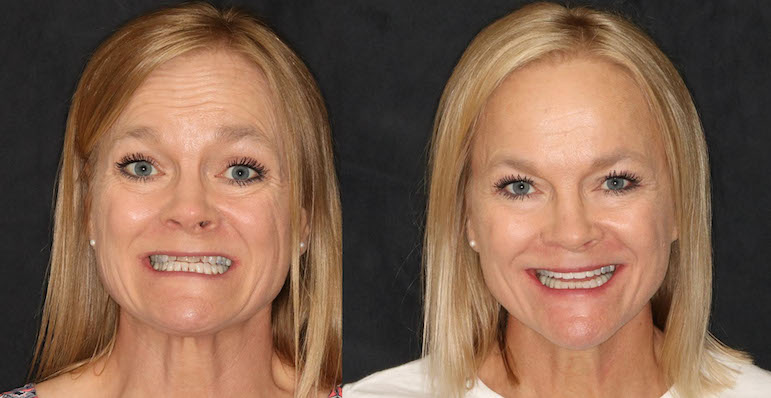This marketing-style photo features a before-and-after comparison of a middle-aged Caucasian woman with blonde hair and blue eyes, highlighting the improvements from cosmetic dental work. Both images show her from the neck up against a black background. In the left image, depicted as the 'before' shot, she wears a wide smile that reveals her yellowish and uneven upper teeth. Her long, straight blonde hair is parted slightly off-center and tucked behind her ears. She has visible wrinkles on her forehead and around her face, and is wearing pearl earrings. 

On the right side, the 'after' image showcases the same woman smiling broadly, now with bright, white, even teeth, indicative of significant dental treatment. Her hair remains parted the same way, and her blue eyes are accentuated with heavy mascara as in the 'before' picture. The wrinkles on her forehead and face have been noticeably reduced, and her overall appearance suggests a more youthful and rejuvenated look. The contrast between the two images clearly illustrates the transformative effects of cosmetic dentistry, potentially aimed at highlighting a dentist's ability to enhance a patient's smile and overall facial appearance.